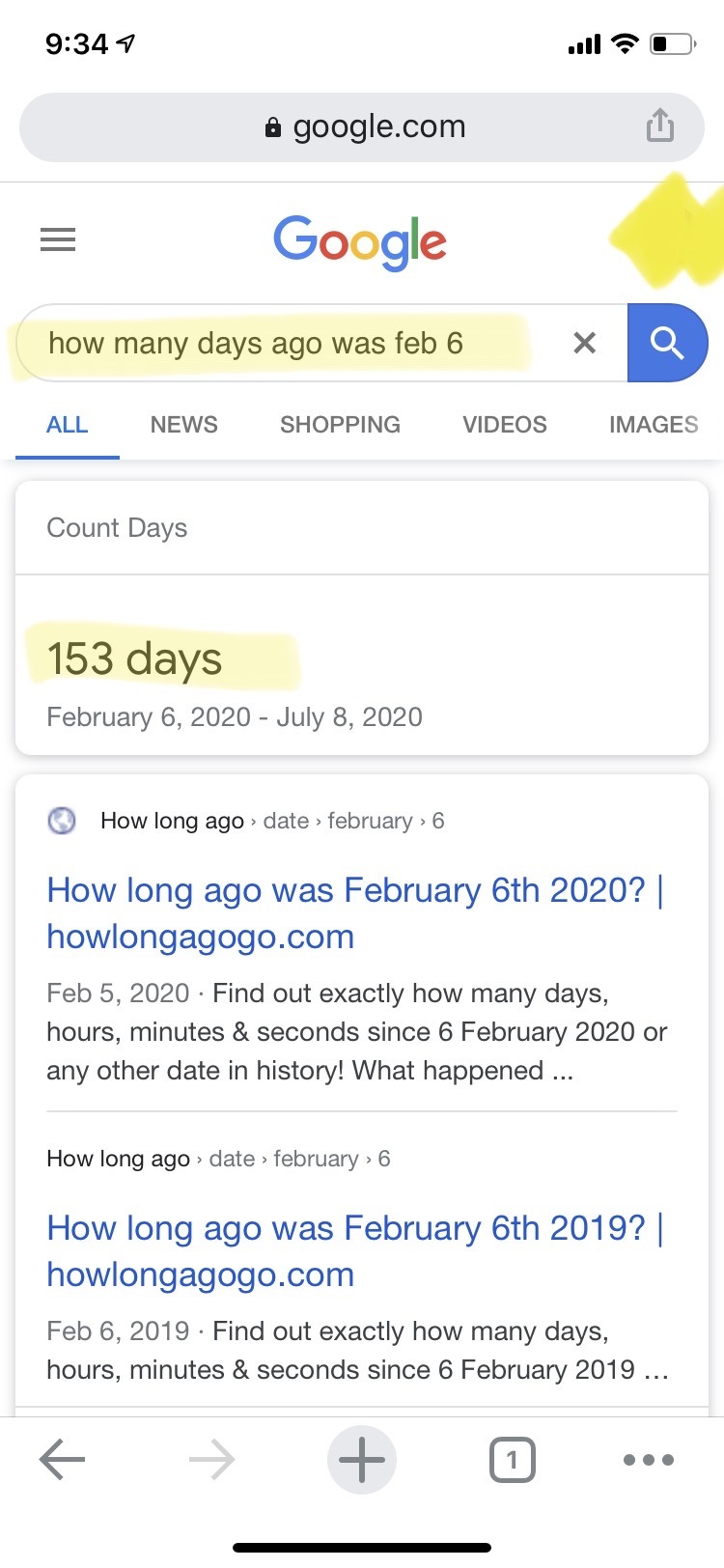A screenshot of a Google search displayed on a mobile phone. The phone's status bar includes a black "9:34" on the left and a Wi-Fi icon on the upper right-hand side, with the battery level below half. Below the status bar is a gray address bar featuring a lock symbol, "google.com" in black, and an upload icon. The center of the screen shows Google's multicolor logo, flanked by the three-line menu icon on the left and an unclear yellow scribble on the right.

The first search box is highlighted in light yellow and displays the query, "how many days ago was February 6th," including an 'X' in the magnifying glass to the right of the input. Below this are category tabs: "All" in blue, with "News," "Shopping," "Videos," and "Images" in gray; the "All" tab is underlined with a blue line.

The main search results show:
1. Count days result in gray showing "153 days" highlighted in light yellow, followed by the timeline "February 6th, 2020 - July 8th, 2020."
2. An Earth icon with the phrase "how long ago" next to it, followed by date particulars.
3. Two primary organic search results with linked titles in blue, descriptions in gray, and dividers between them.

The first result title is "How long ago was February 6th, 2020 | howlongago.com," followed by brief description text, and a gray divider. The second result follows similarly with the title "How long ago was February 6th, 2019 | howlongago.com."

At the bottom of the screenshot, navigation options include a left-facing arrow in darker gray, a right-facing arrow in lighter gray, a circle with a darker gray plus sign, a gray box with the number "1" and three circles, and a black line in the middle of the screen.